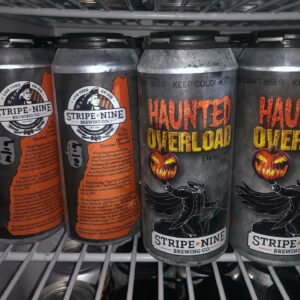The image depicts the interior of a store fridge with a white rack and metal bars, showcasing the middle shelf filled with cold beverages. There are four metallic silver cans prominently displayed. The two cans on the left feature a logo with a George Washington-like figure and an American flag background, with an orange silhouette of New Hampshire and text that reads "Stripe 9." The two cans on the right belong to the same brand, Stripe 9 Brewing Company, but these cans are labeled "Haunted Overload." They have a vibrant orange and yellow design with an illustration of a headless horseman on a black horse, holding up a sinister-looking jack-o-lantern. The fridge shelf also shows the typical black plastic pack tops found in six or eight packs.